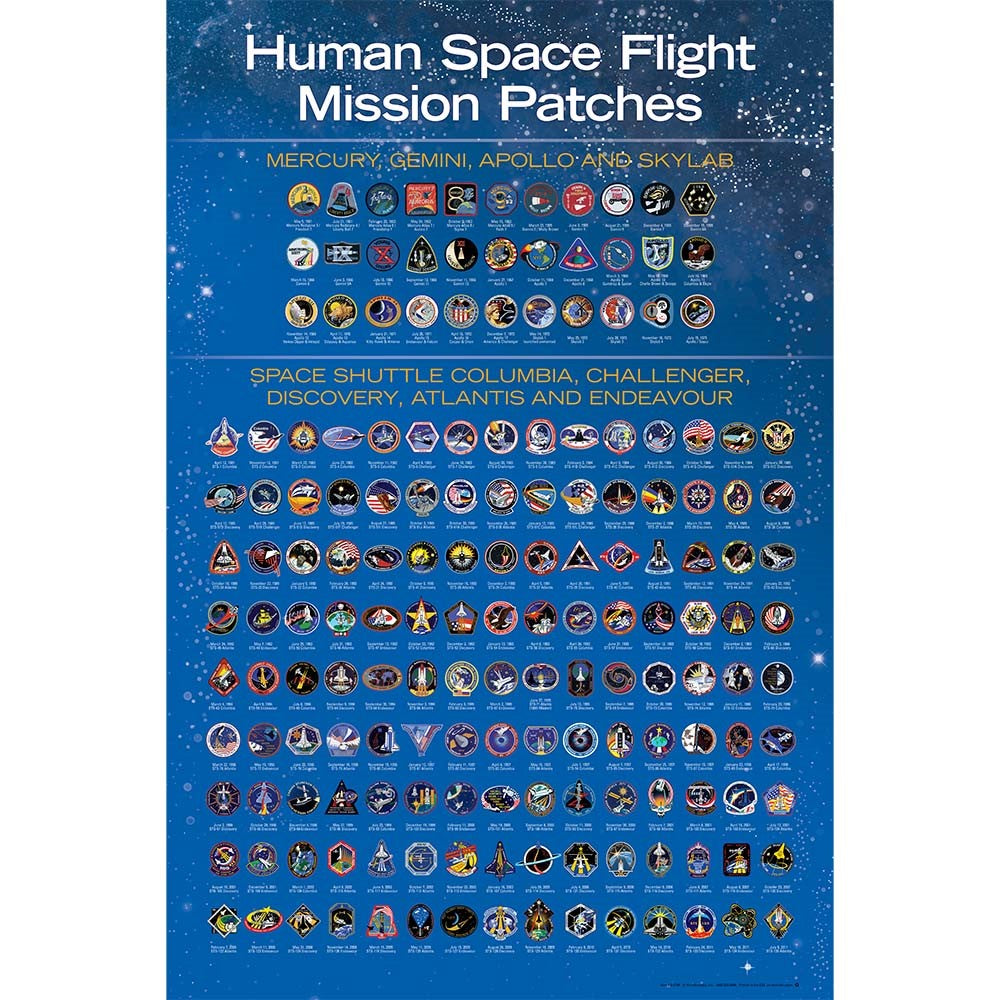The image is a large, rectangular poster measuring approximately 6 inches high by 3 to 4 inches wide. The background features a gradient transitioning from a dark blue at the top to a regular blue towards the bottom, adorned with light gray circles, stars, and constellations scattered across it. At the top center, two lines of bold white print are underlined in blue. The text reads "Human Space Flight Mission Patches," followed by "Mercury, Gemini, Apollo, and Skylab" in gold print. Below this header, the top section of the poster showcases three rows of emblems, each row containing 11 patches of varying shapes like triangles and squares, with small text beneath each patch.

A horizontal light blue line divides this top section from the bottom portion of the poster. Below this line, another gold text header reads "Space Shuttle Columbia, Challenger, Discovery, Atlantis, and Endeavor." The bottom section contains nine rows of additional patches, each uniquely shaped, sized, and colored, with corresponding text underneath them. The overall design is rich in detail and color, illustrating a comprehensive array of human spaceflight mission patches.